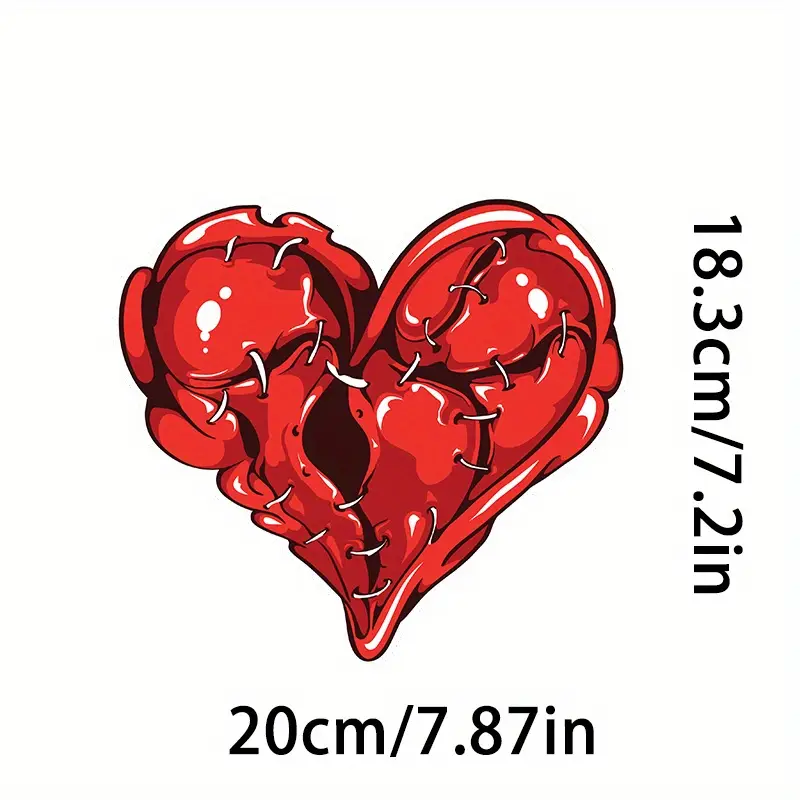This digitally-inked and colored illustration features an organic, irregularly-shaped heart, portraying a vivid, fleshy appearance with a glossy texture. The heart is segmented into three distinct sections: one at the bottom, one on the upper right, and one on the upper left. These segments are held together by white stitches with black outlines, giving the impression that the heart is being carefully stitched or tied together to prevent it from opening up. The entire heart is set against a solid white background, emphasizing its red and dark red hues, further highlighted with white accents to mimic the look of wet flesh. Dimensions are marked in bold black text: on the right side, it states "18.3 cm / 7.2 inches" vertically, and along the bottom, "20 cm / 7.87 inches" is displayed horizontally.